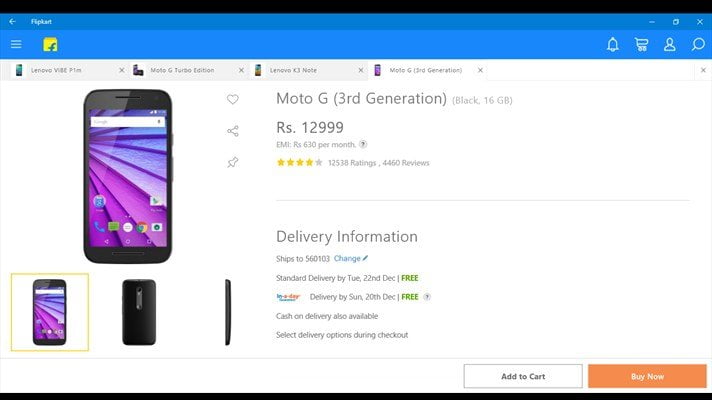The image depicts a website interface showcasing a listing for a Moto G (3rd Generation) Black 16GB smartphone, priced at ₹12,999. The top and bottom edges of the webpage are framed by black rectangles. At the top, the navigation section includes a blue rectangle featuring a back arrow, a pair of horizontal parallel lines, and a folder icon. There are also icons for notifications: a bell (notifications), a shopping cart, and a person (account).

The webpage is cluttered with four open tabs, and the current focus is on the fourth tab. The product listing highlights that the Moto G (3rd Generation) phone has received numerous ratings, with an average of 4 out of 5 stars rendered in yellow. The review count exceeds 12,000. 

Delivery options indicate that the product is available with free shipping and an estimated delivery date by Tuesday, the 22nd. Prominent call-to-action buttons are displayed in orange for "Buy Now" and in white for "Add to Cart," making it convenient for users to make a purchase.